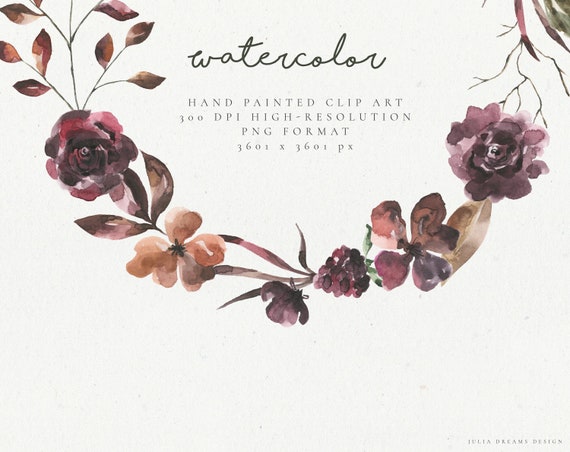The image depicts a detailed watercolor painting of flowers arranged in an upside-down arc or U-shape, stretching from the top left corner, through the center, and up to the top right corner. The delicate flowers exhibit a mix of purple, red, orange, and green hues, with visible stems and leaves. The white background enhances the intricate watercolor design. Prominent text at the top of the image features "Watercolor" in cursive, followed by "Hand-Painted Clip Art, 300 DPI, High Resolution, PNG Format," and "3601x3601px" in a regular font. In the bottom right corner, there's an artist's signature, although it's too small to be clearly read.